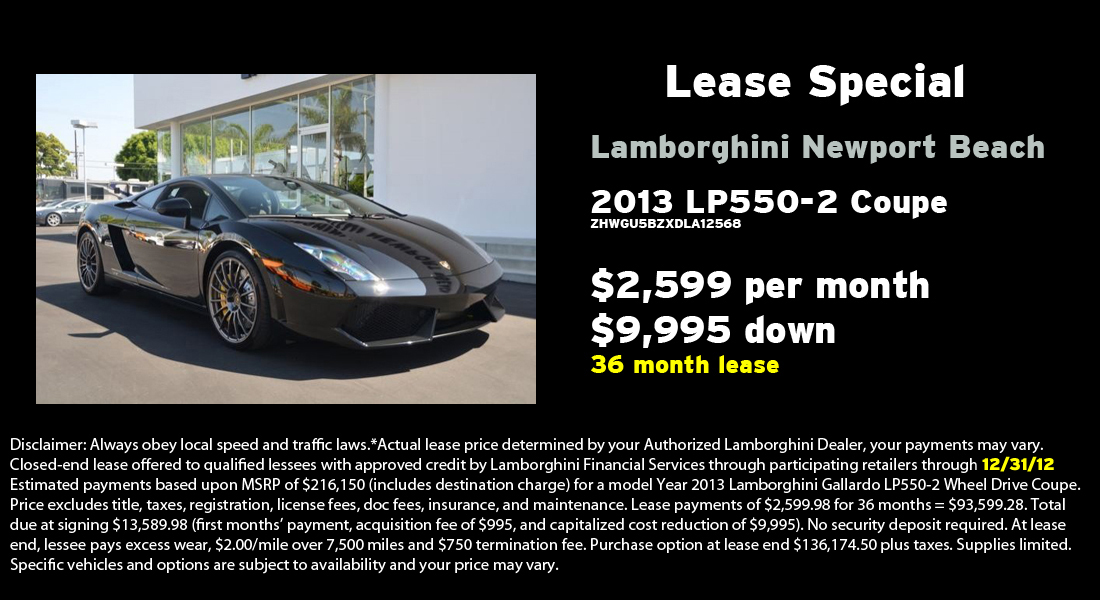This digital advertisement features a special lease offer for a Lamborghini from Newport Beach. The ad's background is entirely black, with white and yellow text prominently displayed on the right side. At the top, it reads "Lease Special" in white letters, followed by "Lamborghini Newport Beach" in light blue and the model "2013 LP 550-2 Coupe" in white. Below this, the payment details are clearly spelled out: "$2,599 per month with $9,995 down" in white text, and "36-month lease" in yellow letters. The bottom third of the advertisement contains a long disclaimer in fine print that includes warnings about obeying local traffic laws and other leasing conditions. 

On the left side of the ad is an image of the sleek, dark gray Lamborghini, facing towards the lower right. The car is elegantly designed with smooth lines and steel rims, parked in front of the dealership. The background showcases the Lamborghini dealership, with additional cars visible, emphasizing the premium setting. The ad concludes with a note in yellow lettering, stating that the offer is "valid through 12-31-12."